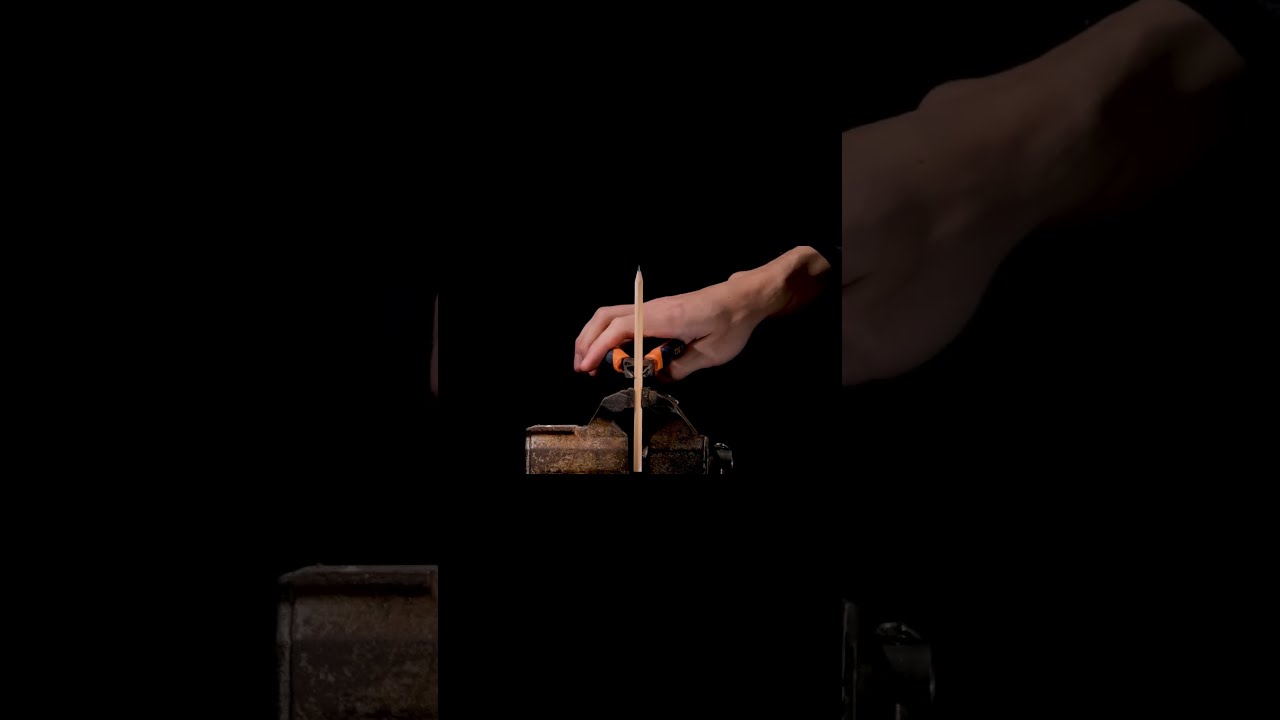In this vertically-oriented image with a completely black background, a Caucasian right hand is centrally positioned, holding a pair of black-handled and orange-tipped pliers. These pliers are gripping a light brown wooden pencil, which is being held vertically. The hand and the pencil are both captured in vivid detail. The pencil appears to be ready to be cut by the pliers. Below the pencil, there's a rusted, brown metal clasp adding to the composition. On the left side of the image, a brown box rests on the surface beneath the setup. The overall gaze zeroes in on the act of imminent cutting or snapping of the pencil by the pliers, with stark contrast provided by the dark background.